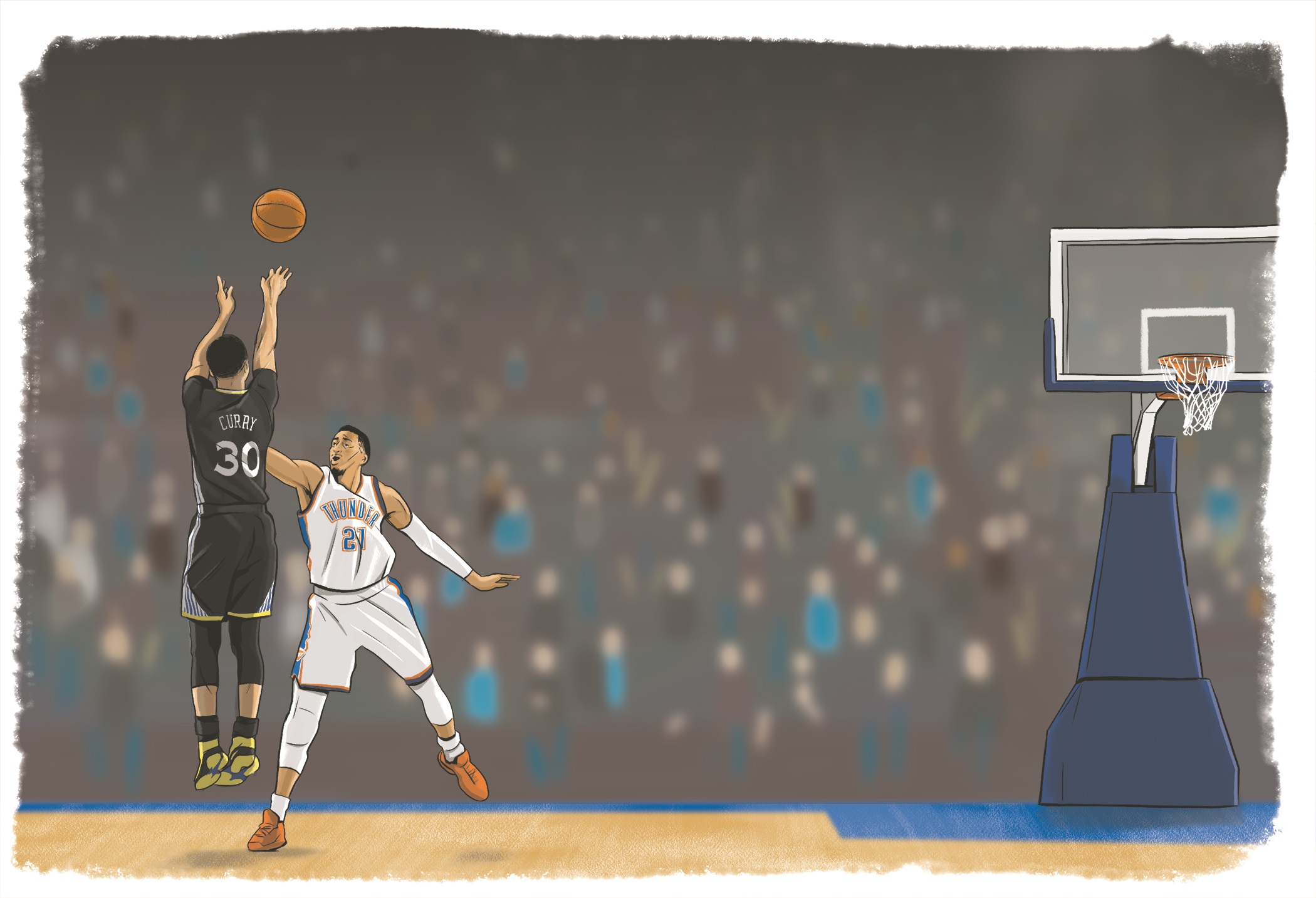This image portrays a stylized, somewhat cartoony yet realistic scene reminiscent of a comic book or graphic novel style, depicting a tense moment in a basketball game. On the left, player number 30, identified as Curry, is mid-shot, having just released an orange basketball. He is dressed in an all-black uniform with gray and gold accents, including gold shoes. Opposing him is a player in a white jersey, seemingly numbered around 21 to 29 and labeled "Thunder," attempting to block the shot with an outstretched arm. This player wears white knee pads and orange shoes, with a white compression sleeve on one arm. The setting includes a smudged, smoky background populated by indistinct, oval-headed spectators in dispersed blue and black shirts, blurring into the stadium seats. The basketball hoop, featuring a clear backboard outlined in white, stands on a blue pedestal with a blue-bordered tan floor beneath, anchoring the dynamic scene.